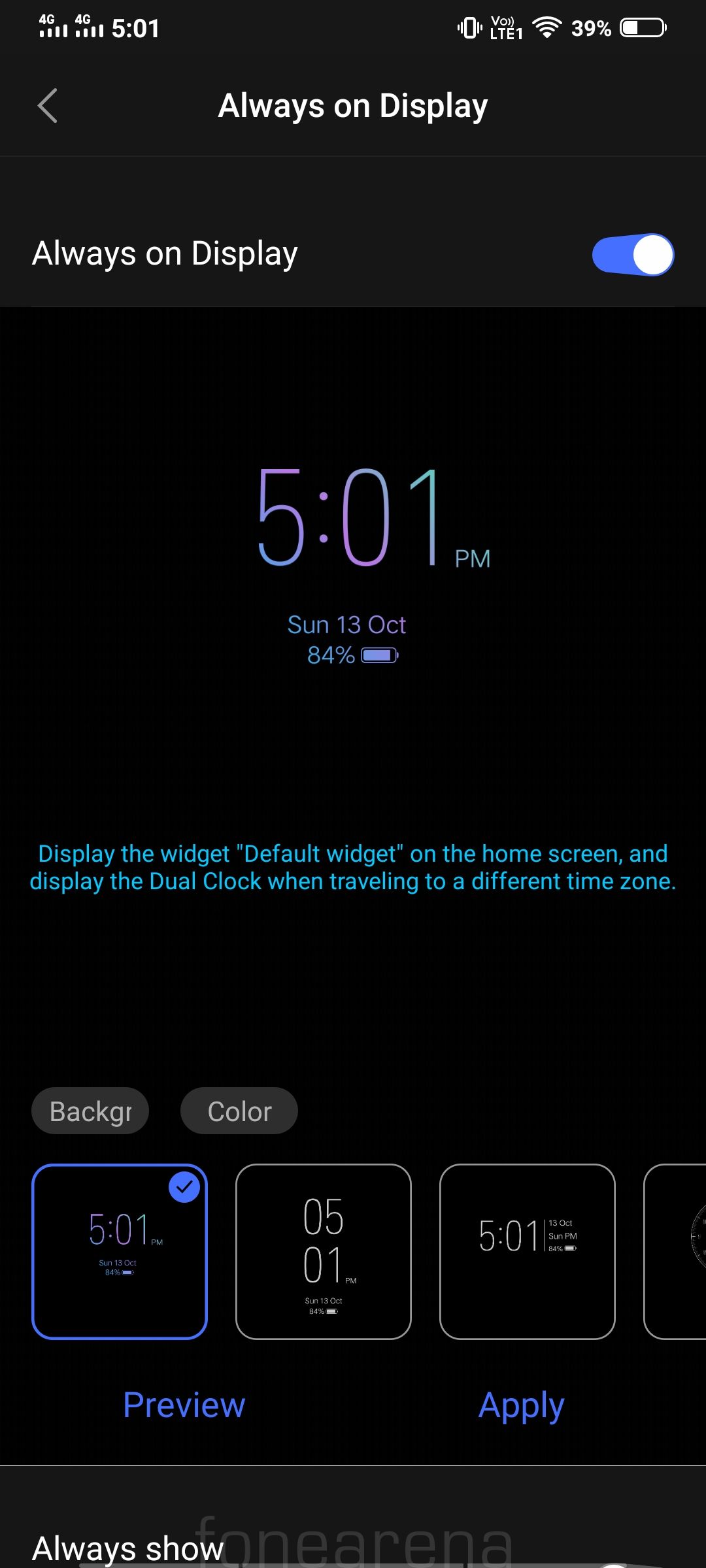A screenshot from a cell phone captures the time at precisely 5:01 PM, displayed in the upper right-hand corner. The image has an 'Always On Display' interface featuring a predominantly black background. The top half is a lighter shade of black, contrasting with a darker black in the bottom section. 

The time "5:01 PM" is prominently highlighted in vibrant colors; the "5" and the colon ":" are purple, transitioning to an aqua green for the "0", "1", and "PM". The fonts and symbols on the display are entirely white, including a back arrow situated below the 'Always On Display' label on the left side of the screen. To the right of this label is a large gap followed by a toggle button set to the 'on' position. The meticulous contrast and vibrant accents give the image a visually striking appearance.